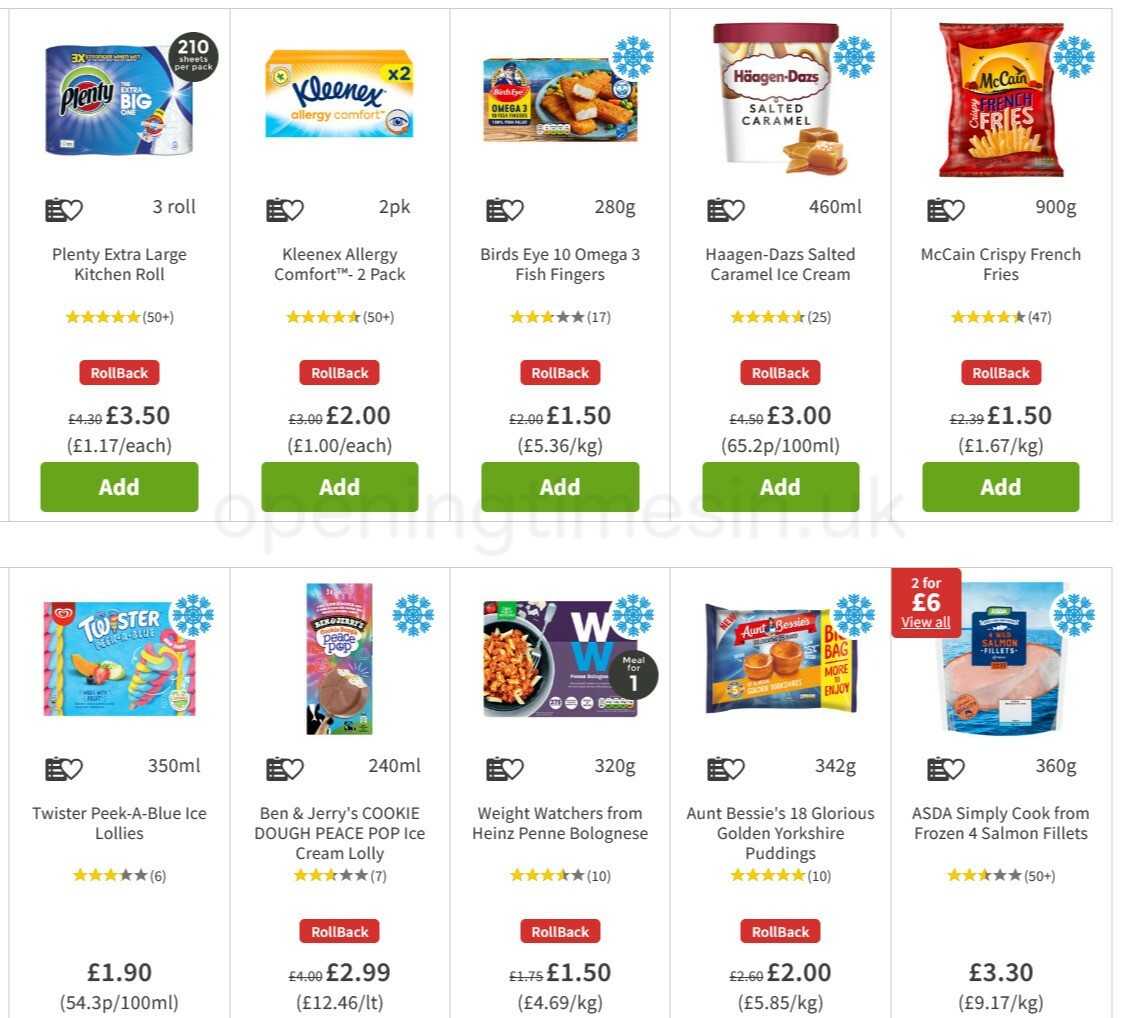Here is a more detailed and polished caption for the grocery store image:

---

This appears to be a digital catalog page from a grocery store, featuring two horizontal rows of grocery items. Each product is presented with an accompanying image, a description, and a price listed in pounds, indicating a UK-based store. Notably, each item image includes a prominent red button labeled "rollback" in white text, hinting at a potential discount or promotional offer. Below each product image, there is a green rectangular box displaying the word "add" in white, allowing customers to easily add items to their shopping cart. 

The first row showcases the following items from left to right:
1. **Plenty Extra Large Kitchen Roll** – A package of paper towels ideal for household cleaning and spill management.
2. **Kleenex Allergy Comfort Tissues (2 Pack)** – Soft tissues designed to provide relief for those with allergies.
3. **Birds Eye 10 Omega 3 Fish Fingers** – Breaded fish fingers enriched with Omega-3, perfect for a quick and nutritious meal.
4. **Haagen-Dazs Salted Caramel Ice Cream** – A luxurious and creamy ice cream with a rich salted caramel flavor.
5. **McCain Crispy French Fries** – A bag of crispy french fries that cook to perfection, ideal for a crunchy side dish.

In the second row, the following items are displayed:
1. **Twister PIKA Blue Ice Lollies** – Vibrantly colored ice lollies, offering a refreshing treat for the warmer days.
2. **Ben and Jerry's Cookie Dough Peace Pop Ice Cream Lolly** – A delightful ice cream lolly with chunks of cookie dough, catering to the sweet tooth.

---

This refined caption provides a clear and thorough description of the image, highlighting each product and its key features.